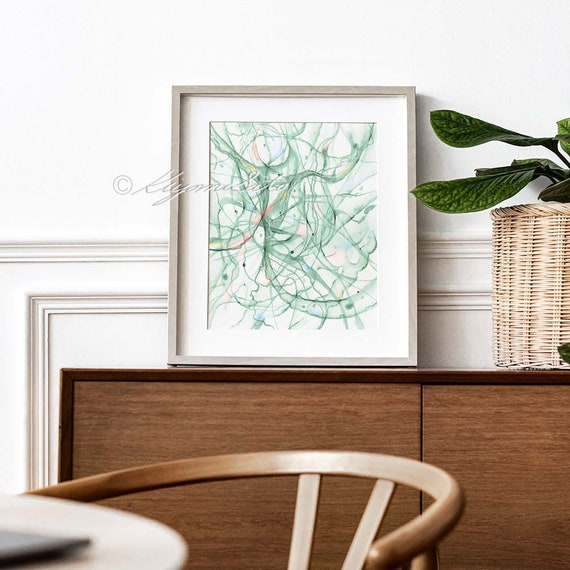In a cozy and well-decorated room featuring white walls with decorative trim, a wooden table stands prominently against the wall. This table, which has two sliding doors, holds a framed piece of abstract art characterized by multiple swirling lines and colors, including green, white, red, and hints of orange. The painting, which has a watermark that is difficult to read but seems to say "copyright Kiyomasito," is propped against the wall, adding an artistic touch to the scene. To the right of the framed art, a wicker-type basket pot contains lush, green leaves, adding a natural element to the arrangement. In the foreground, a wooden chair with a rounded back is positioned next to a round table, also made of wood, creating a warm and inviting atmosphere.